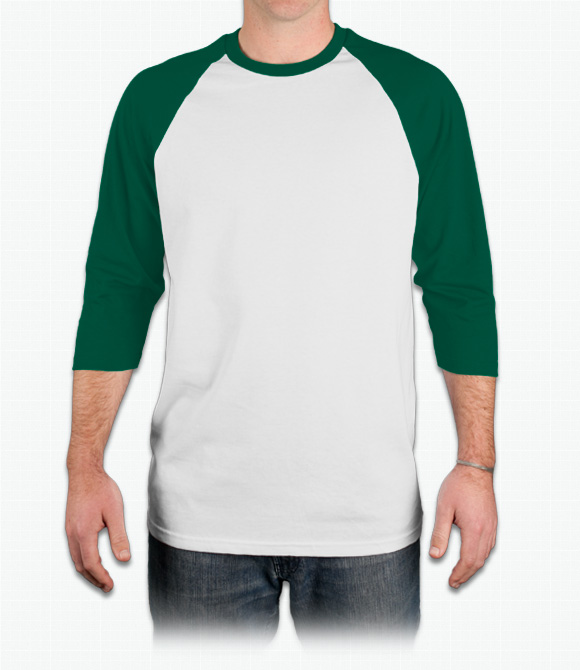The photograph is a carefully staged, full-color image with a pure white background. It depicts a Caucasian male from just below his chin to the top of his thighs, showcasing a white t-shirt with green three-quarter-length sleeves and a matching green collar. The man is dressed in dark blue jeans and has fairly hairy arms, with his hands resting by his sides. Notably, he has a silver band on his left wrist. The positioning of the image and the stark background suggests it is a stock photo, likely for the purpose of highlighting the t-shirt.